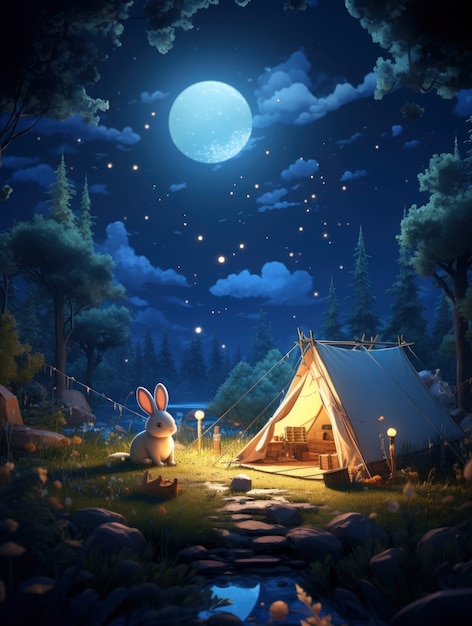This digitally created artwork, scanned for viewing, displays a nighttime campout scene in a vertically oriented rectangle. Dominating the foreground on the left, we find a small, soft-looking white bunny with pink ears seated on a patch of grass. On the right, a beige, triangle-shaped tent is illuminated by soft yellow light from small glowing orbs, possibly lawn ornaments, situated on either side of the tent.

The middle section features a stone path leading down to a small, reflective pond, flanked by scattered rocks and pebbles. In the background, further away and occupying the middle of the scene, lies a larger lake surrounded by a range of trees including prominent pine trees that frame the dark sapphire blue sky.

The sky itself is dotted with stars or glowing fireflies, adding a magical touch, along with light blue-gray puffy clouds and a large luminous moon with hints of blue and gray, casting a serene glow over the entire campsite.